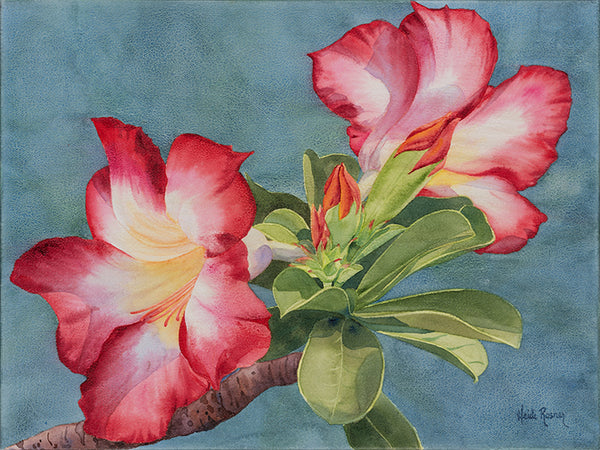This painting, presented on a horizontally-oriented canvas about one and a half times as wide as it is tall, features an elegant and classy depiction of two large tropical flowers with rich magenta petals and light pink interiors. The flowers are situated on a brown wooden stem that extends from the bottom left corner, slightly upward and to the right, terminating in the middle of the image. Between the flowers, you can find an assortment of long, oval-shaped green leaves. One flower, fully bloomed, faces toward the left and the viewer, positioned on the left side of the composition. The other flower, also fully bloomed, is situated in the upper right portion of the painting, facing away and slightly to the right. The background is a dark teal or bluish color, adding a layer of sophistication to the overall scene. Near the bottom right corner of the painting, the artist's signature, "Heidi Rosner," is visible in blue text.